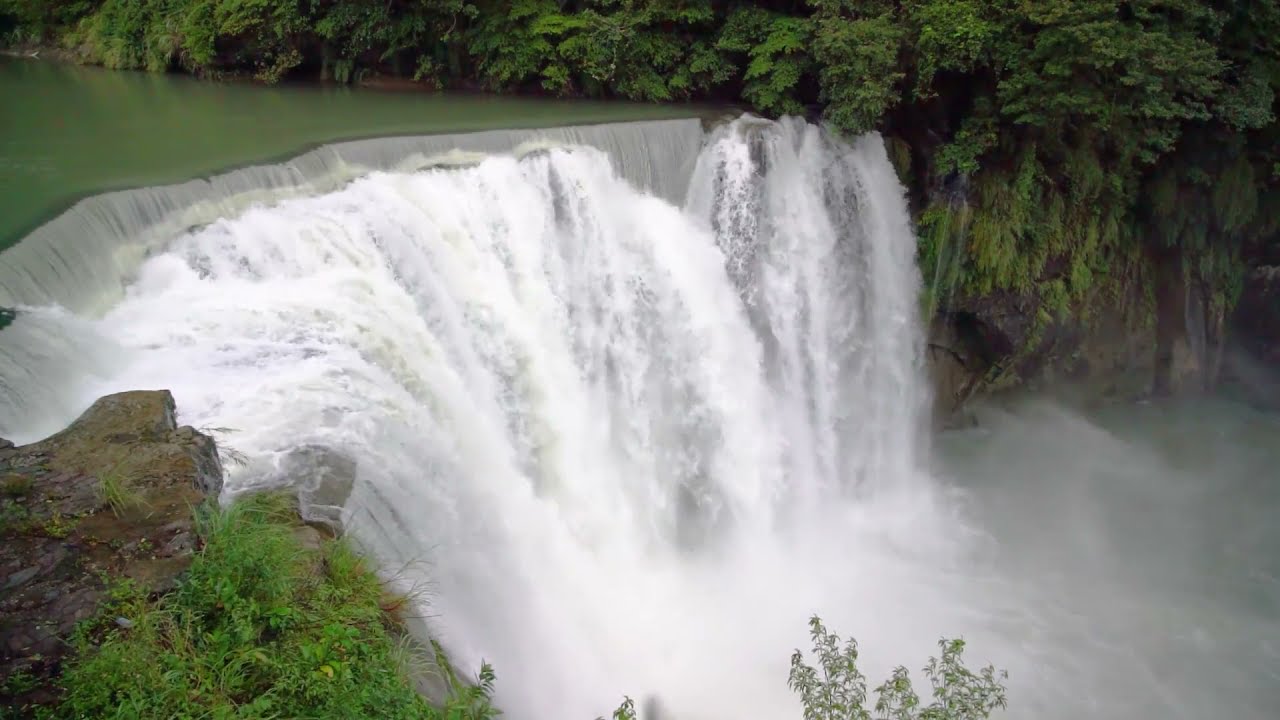This detailed aerial view captured by a drone shows a mesmerizing waterfall descending from a small river that snakes through a lush forest. The image is a wide, horizontal rectangle, with the waterfall starting near the upper left and curving gracefully across the frame before dropping past the center. This high-angle shot reveals the still, green water at the river's surface, likely reflecting the dense foliage and vibrant greenery surrounding it. 

As the water reaches the cliff edge, it cascades down steeply, turning white from the speed and crashing with torrential force into the misty abyss below. This mist rises and creates a foggy, cloud-like effect at the waterfall's base, obscuring the view of the pool it feeds. The entire scene is enveloped in dense trees and shrubs, adding to the natural beauty and secluded feel of the area. 

Overall, the image evokes a sense of powerful but serene natural beauty, reminiscent of a smaller version of Niagara Falls, complete with vibrant green hues and dynamic water movement.